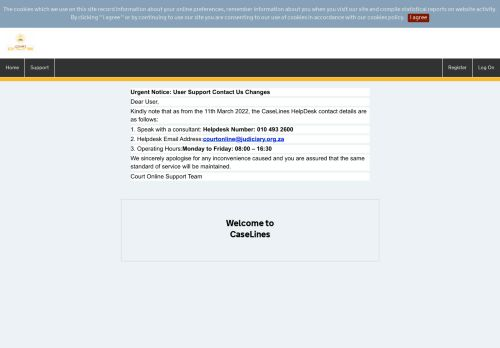**Caption:**

The screenshot features a light blue background with a structured layout. At the top, a blue rectangle contains important information, followed by a red rectangle with the text "I agree" prominently displayed in white. Below, a blue navigation bar includes options labeled "Home," "Support," "Register," and "Logout," plus an additional white square icon.

An urgent notice follows, addressed to users. The message begins, "Dear User, kindly note" and informs the reader about changes effective from March 11th, 2022. The text highlights updated support contact details for the CAST line's help desk:

1. **Speak with a Consultant:** A bolded "Help Desk Number" is followed by a phone number.
2. **Help Desk Email Address:** The email address is highlighted in blue.
3. **Operating Hours:** In bold, the notice states that the help desk is operational from Monday to Friday, 8:00 AM to 4:30 PM.

Additional details are provided further in the notice.